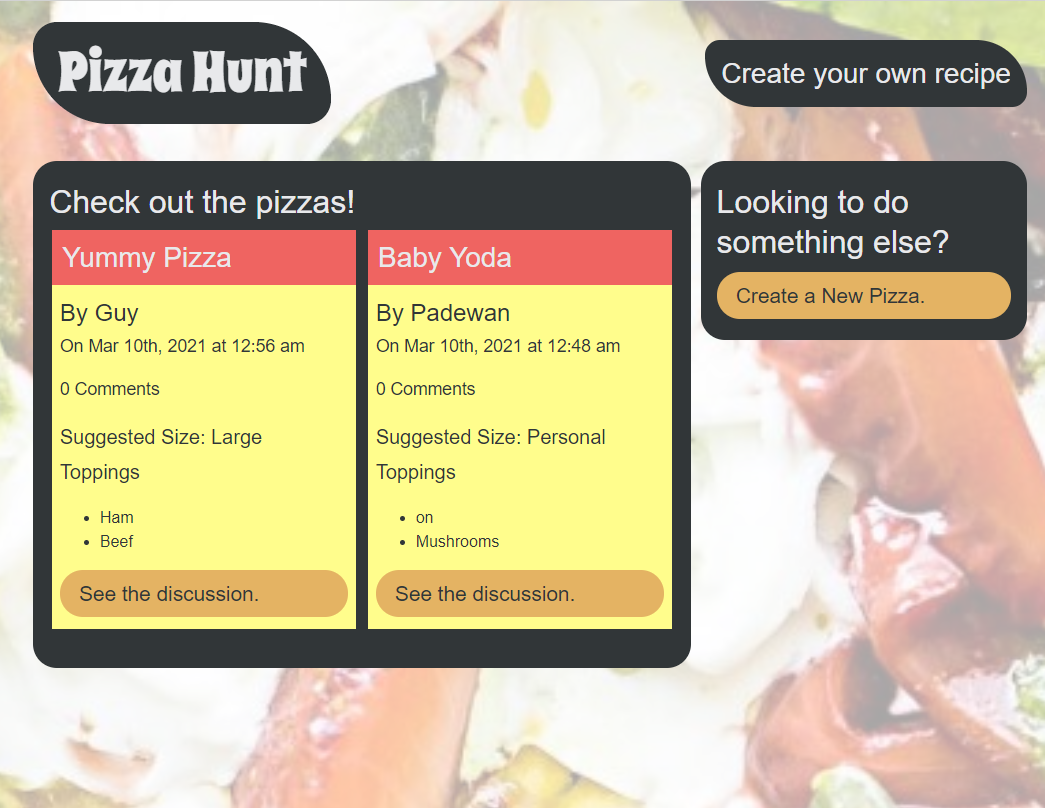The screenshot captures the homepage of Pizza Hunt's website. Dominating the background is a blurred close-up photograph featuring vibrant pizza toppings in shades of red, white, and yellow. This appetizing image sets the tone for the page's content. 

In the upper left corner, the Pizza Hunt logo is prominently displayed in a light font against a black, irregular, rounded rectangle, adding a touch of branding to the site. On the opposite side, in the top right corner, a call-to-action text reads "Create Your Own Recipe," inviting visitors to personalize their pizza experience.

Beneath this, two distinct black boxes serve as focal points for the page's interactive features. The larger box on the left promotes custom-created pizzas with the header "Check Out the Pizzas." Within this section, two pizzas are highlighted with individual descriptions.

The first pizza, "Yummy Pizza," was crafted by Guy on March 10, 2021, at 12:56 a.m. This creation, which has received zero comments, is recommended in a large size with ham and beef as toppings. A yellow pill-shaped button below reads, "See the Discussion."

To the right of this, "Baby Yoda," another pizza created by Padawan on March 10, 2021, at 12:46 a.m., is displayed. This custom pizza, like the previous one, has not garnered any comments. It is suggested as a personal-sized pizza with mushroom toppings. Similarly, a yellow pill-shaped button prompts users to "See the Discussions."

Adjacent to this section is a smaller black box with the heading "Looking to Do Something Else." Below this, a gold pill-shaped button encourages users to "Create a New Pizza," offering an easy pathway for customization.

Overall, the layout is dynamic and user-friendly, enticing users to explore and engage with the various pizza creation options provided by Pizza Hunt.